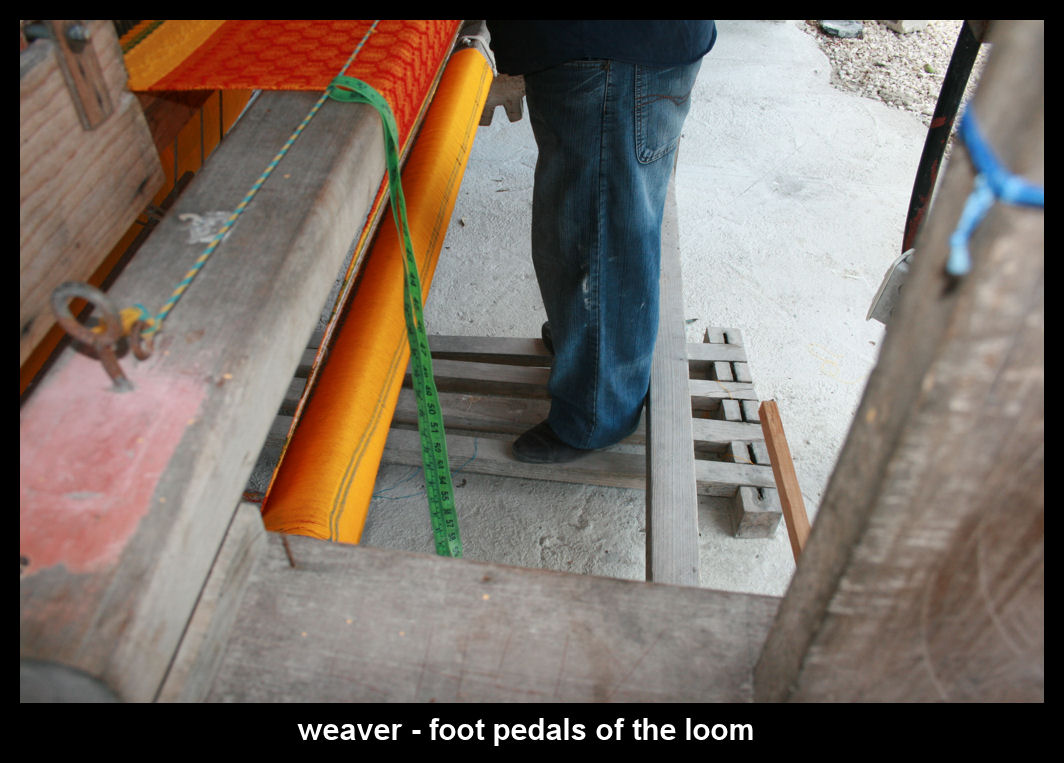In this detailed photograph, only the bottom half of a person is visible as they operate an outdoor loom. The individual, dressed in a dark blue shirt, baggy blue jeans, and black shoes, stands on wooden slats positioned over a concrete surface. The loom, constituted of wooden beams, holds vibrant orange, red, and yellow threads being woven into material. A green measuring tape dangles from a bungee cord stretched across the loom. A pole with a piece of blue fabric tied around it stands to the right, beneath which lies a shelf with a rusty nail. Behind the person, rocks and gravel can be seen, adding to the rustic outdoor setting. The image has a black border, with the bottom strip thicker and displaying the caption "Weaver dash, foot pedals of the loom" in white lowercase letters.